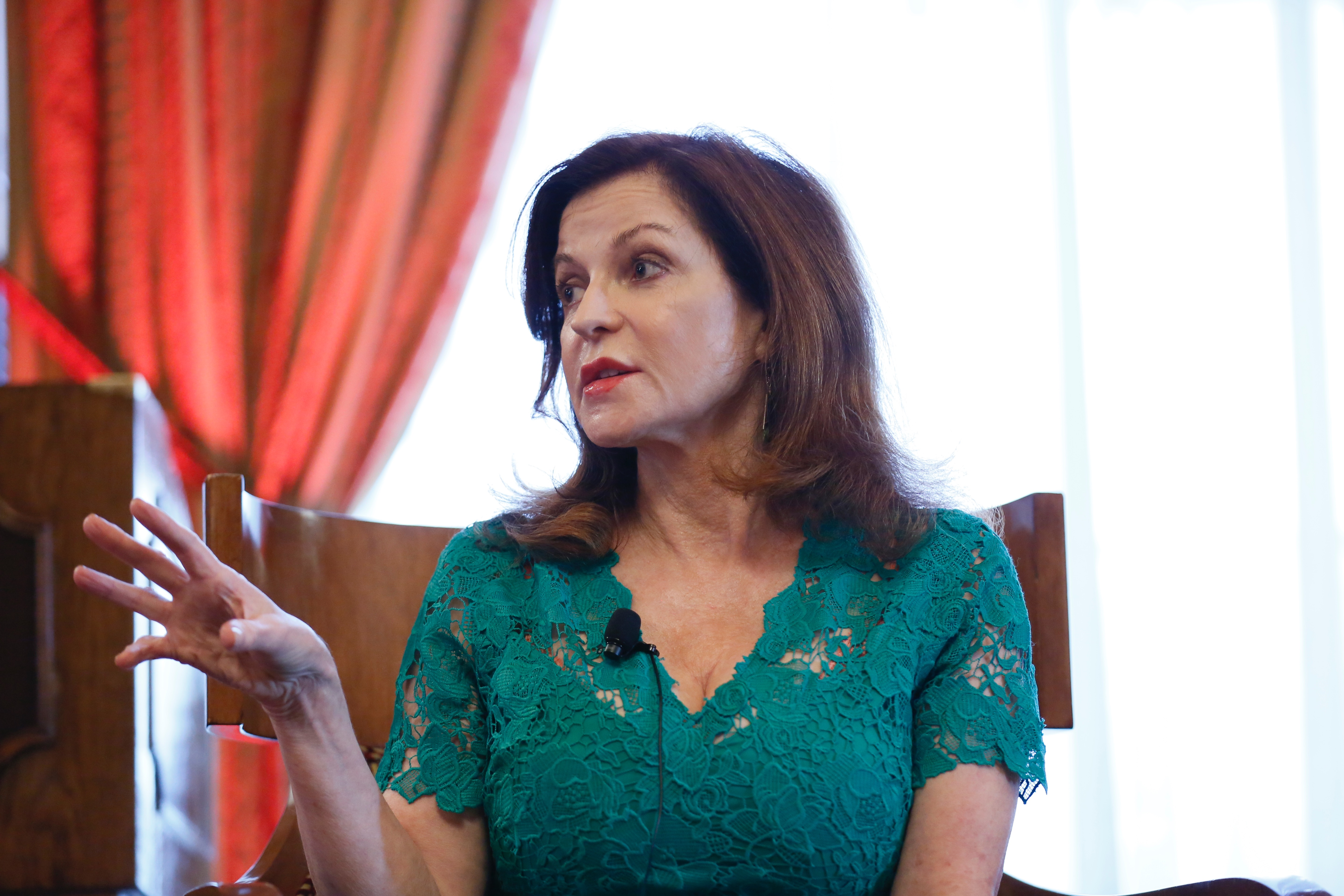This detailed image features a woman seated in the center of the frame, her body facing towards the camera while her head and eyes are turned to the left, as if engaged in conversation. She has reddish-brown hair that falls slightly past her shoulders and is wearing a lacy, turquoise-colored v-neck blouse. The intricate lace pattern is a notable detail of her attire. Her left arm is partially visible up to the elbow, while her right arm is raised, with her hand and fingers splayed out, suggesting she is gesturing.

The background is slightly blurred but noticeably bright, indicating daytime. On the left, a red curtain adds a splash of color, while a white, possibly glary curtain or window panel is visible behind her on the right. There is also a structure partially hidden by the red curtain. The entire scene appears to take place indoors, possibly during a meeting. The color palette of the image includes various shades of brown, white, turquoise, tan, maroon, orange, and pink. Notably, the woman's chair has a distinctive round back that wraps around her, adding to the composition of the image.